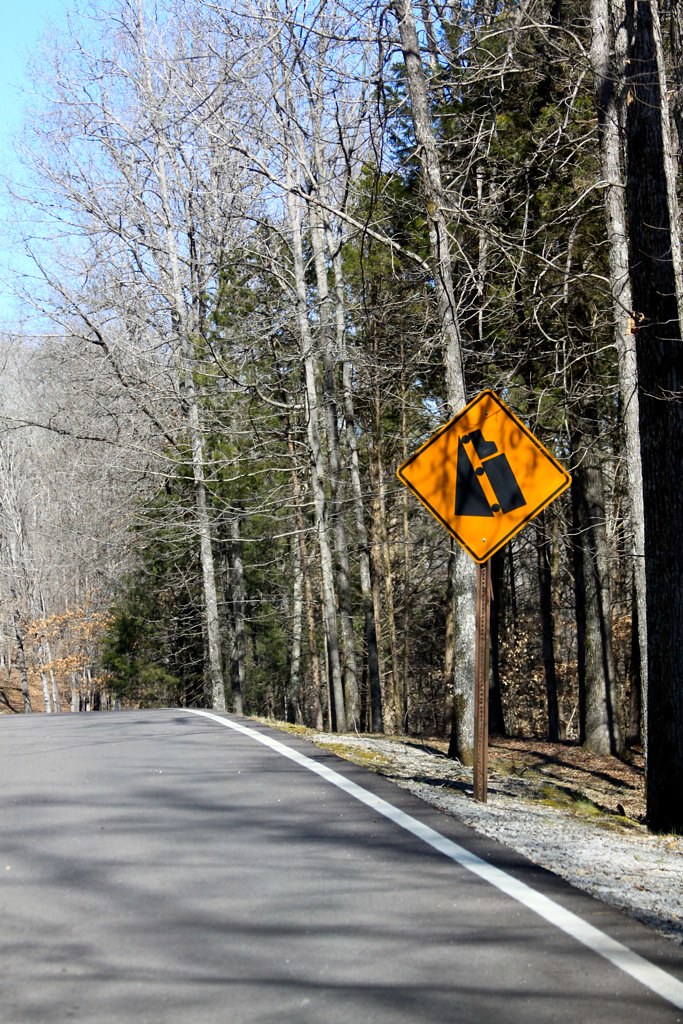A small highway winds through a wooded area, framed by an assortment of trees. Some trees are bare, possibly indicating the onset of fall, while others still retain their green leaves. The image, which appears to be taken from just off the side of the road, features a white line marking the road's edge. A yellow warning sign is visible, cautioning trucks about a steep incline ahead. The shot captures the tranquil, transitional nature of the forested scene, with clear signs of seasonal change.